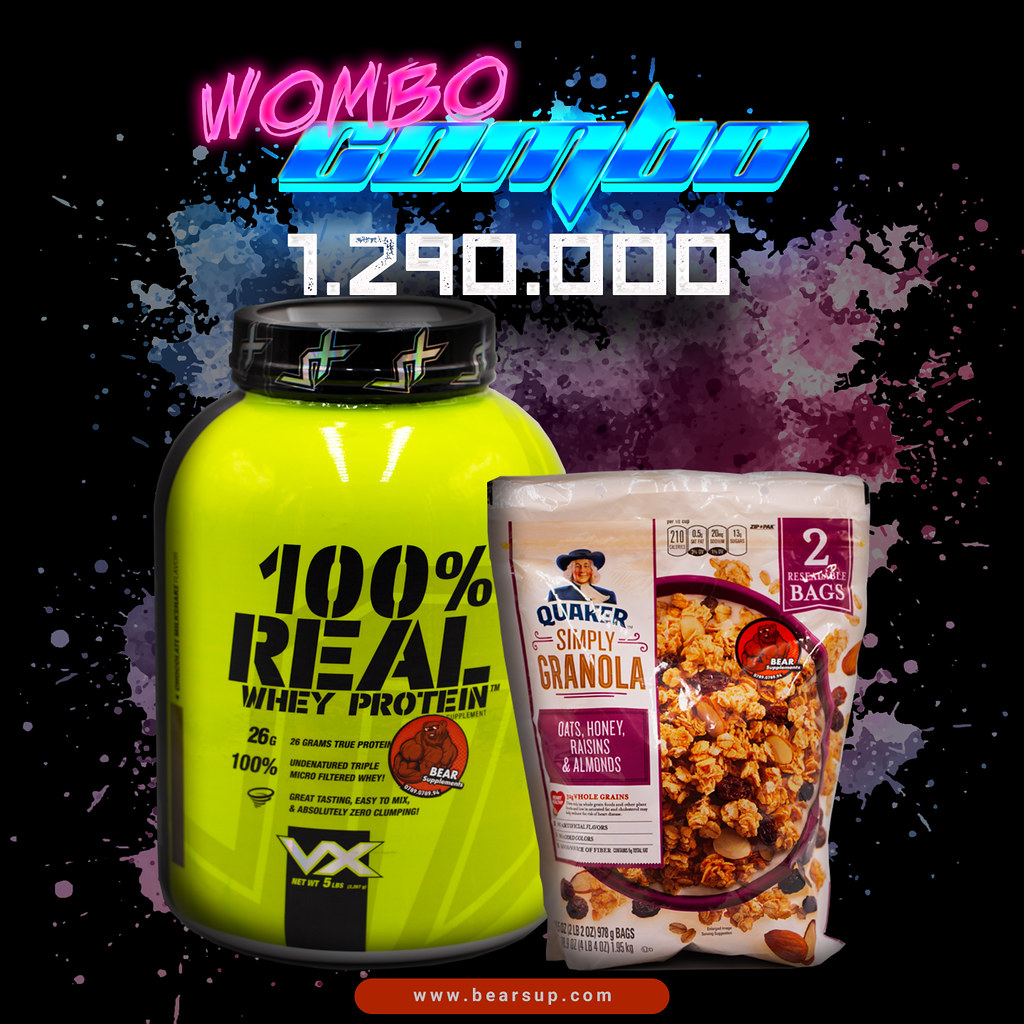The advertisement features a striking black background accentuated by blue and purple paint splatters at the center. Prominently displayed in the foreground left is a large, bright yellow container of VX brand whey protein with a black cap. Bold, black, stencil-styled letters on the container proclaim "100% REAL WHEY PROTEIN," followed by the smaller text, "26 grams true protein," with additional unreadable details.

Adjacent to the right, a Quaker Simply Granola packet sits slightly in front of the whey protein. This small, sealed, foil bag displays an overhead photo of granola mixed with milk, emphasizing its contents of oats, honey, raisins, and almonds.

At the top of the image, the vibrant text "WOMBO" in pink neon is followed by "combo" in a metallic typeface, reading as "WOMBO combo." Below this, in white block numbers, is the figure "1.290.000." At the very bottom center, a watermark reads "www.bearbearsup.com."

This colorful composition combines bold visuals and detailed typography to create a dynamic advertisement.